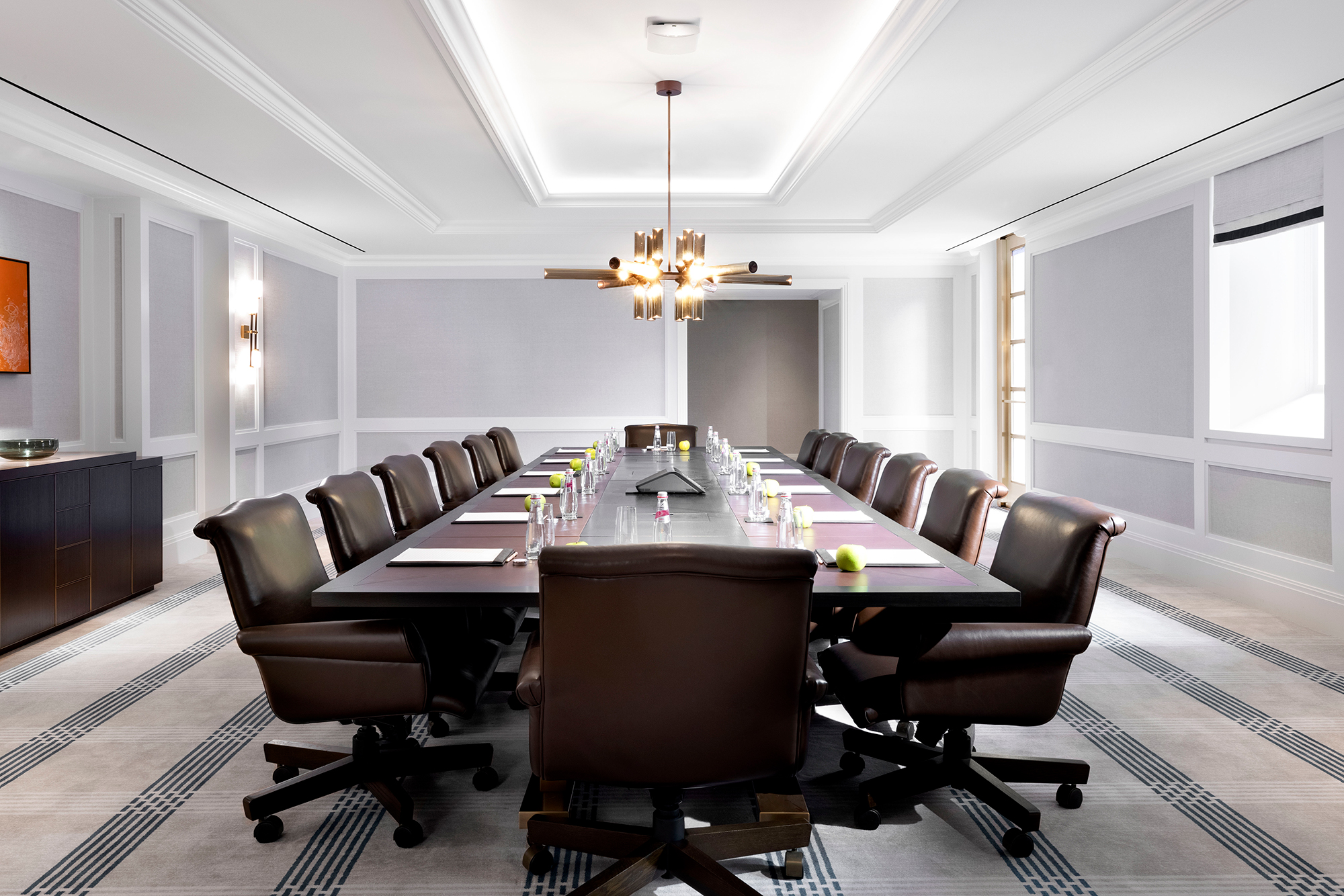The interior of this modern office boardroom is characterized by a long, deep brown mahogany conference table, surrounded by a total of fourteen brown leather rolling chairs, six along each side and one at each end. Positioned in the center of the room is a striking gold-bronze chandelier with crossed pipes or cylinders. Each place at the table is set with a white notepad, a green apple, and a glass bottle of water. The room features gray walls with white accents and a popped white ceiling. On the left side, a brown wood console table supports a TV mounted above it on the wall. The floor is covered in a carpet designed with a black, white, and cream line grid pattern, and there are windows on the right side of the room that allow natural light to filter in.